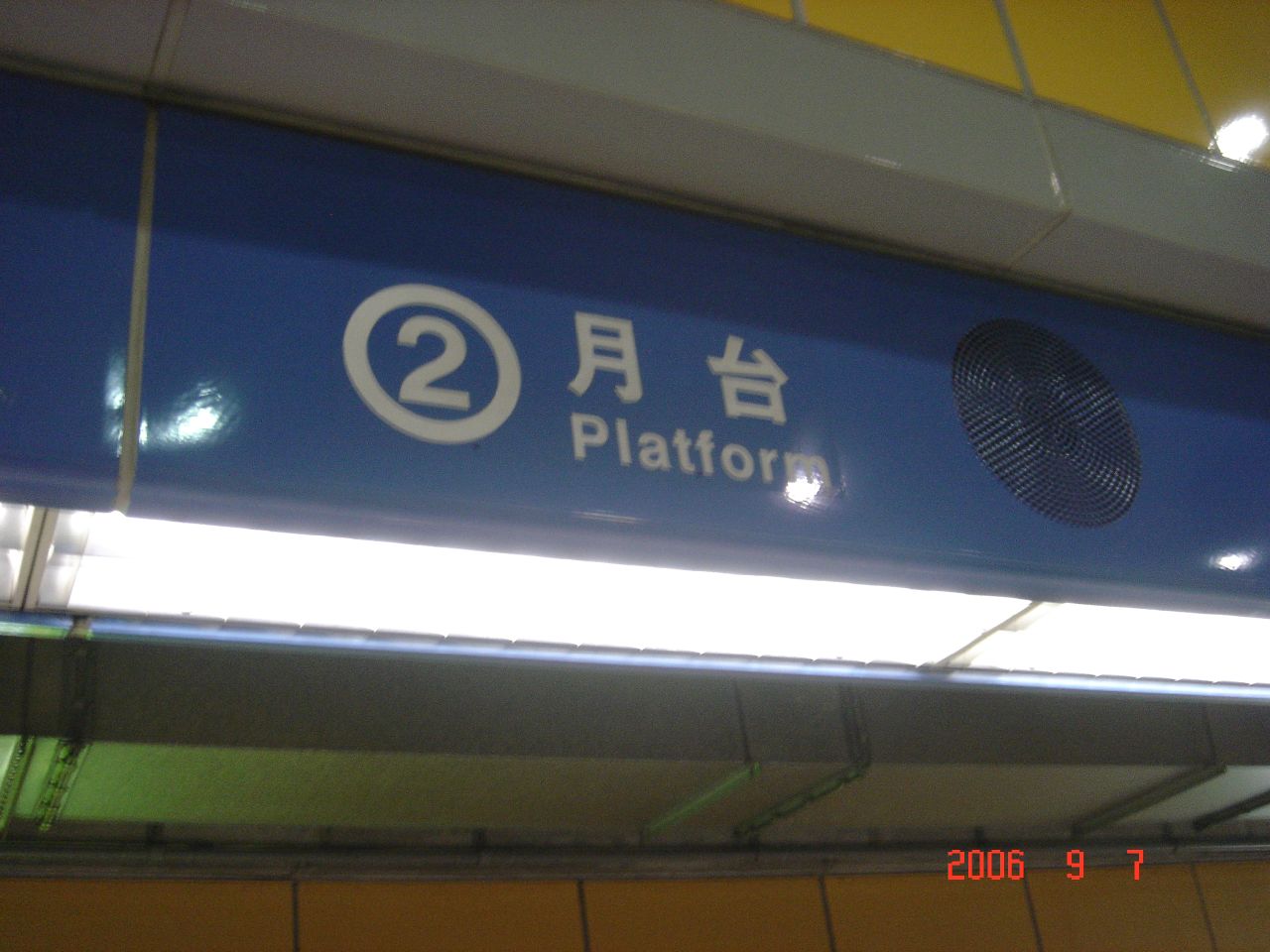A photograph captures a platform that could belong to either a subway, tramway, or railroad. Prominently displayed is a blue sign featuring white characters that read "月台" (Yue Tai), which translates to "platform" in English. The sign also displays the number "2" encircled by a white ring. Above the blue sign, the background wall is painted yellow. At the bottom of the image, the date "2006-9-7" is visible, rendered in an orange-reddish font.